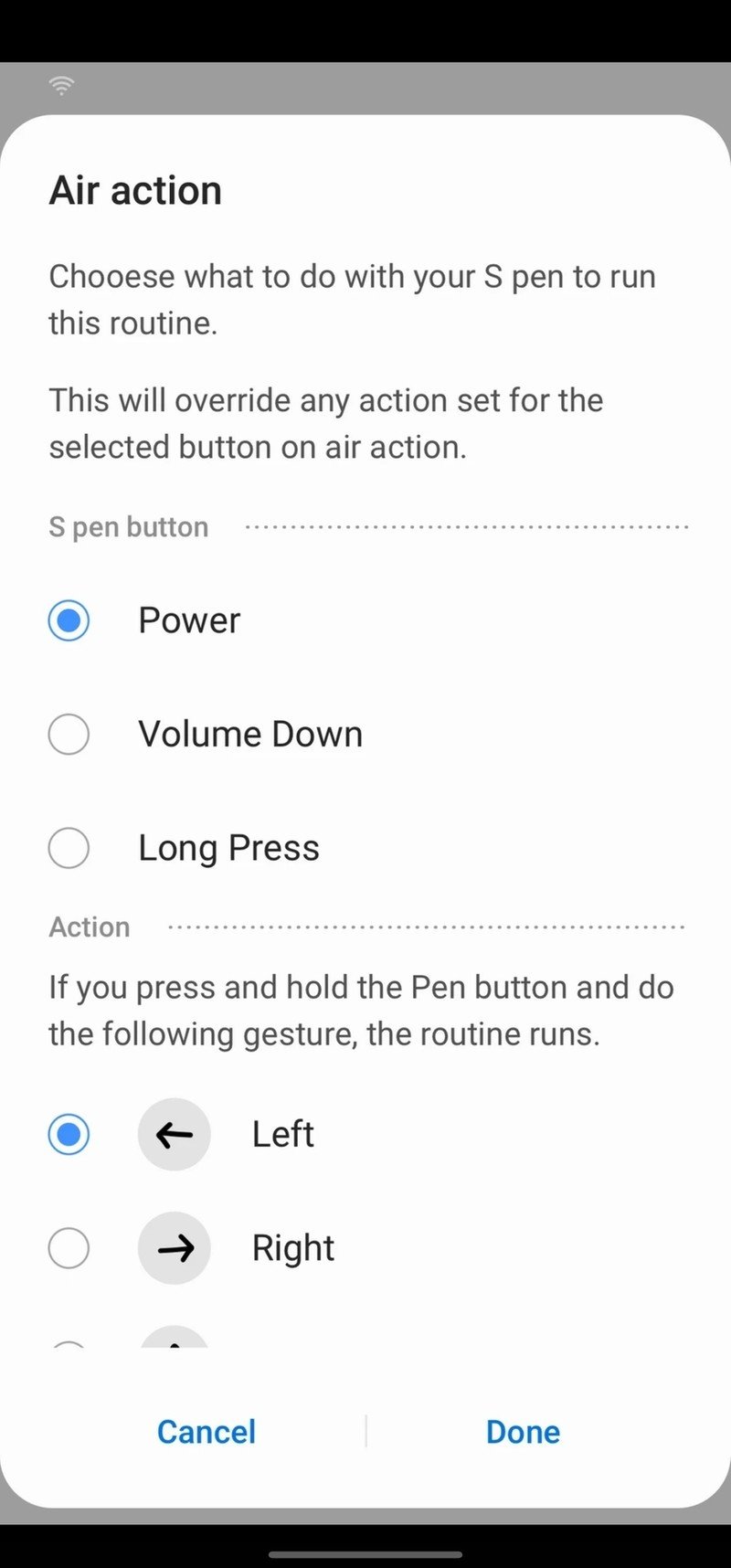The image appears to be a screenshot taken on an iPhone, identifiable by the full bars of the Wi-Fi signal icon displayed at the top left, with a grayish background color in the notification bar. The content of the screenshot highlights a settings page for configuring actions associated with the S Pen.

At the top of the screen, in bold black text, the heading reads "Air action." Directly below, a paragraph states: "Choose what to do with your S Pen to run this routine. This will override any action set for the selected button on Air action." Notably, the word "Choose" is misspelled.

Following this, in light gray text, the label "S pen button" is shown, accompanied by several horizontal dots aligned to the right. 

Below these elements, three options are presented in bubble form. The first bubble is highlighted in blue and labeled "Power." The second bubble is unselected and labeled "Volume down," while the third bubble, also unselected, reads "Long press."

Further down, another category is introduced with the heading "Action." This section explains that if you press and hold the pen button while performing certain gestures, the routine will activate. Two gesture options are displayed in bubbles: the first bubble reads "Left," and the second bubble reads "Right."